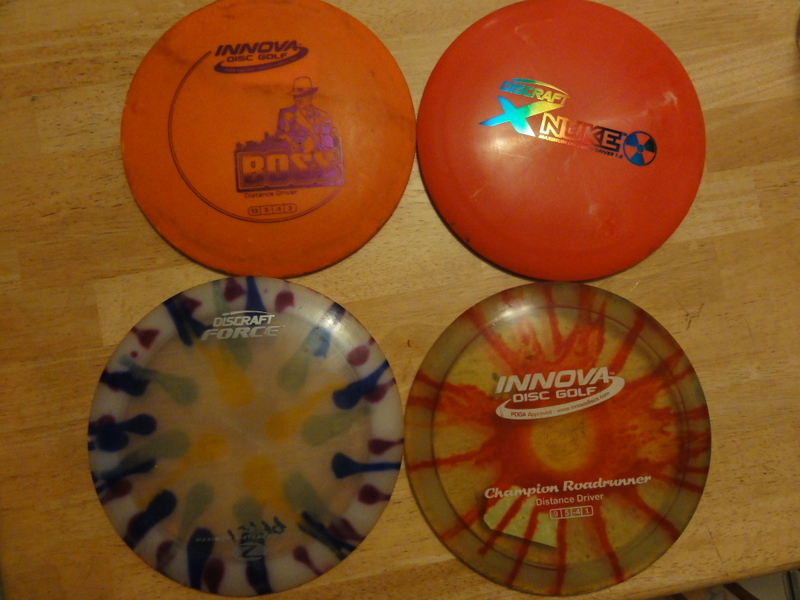This detailed photograph features four disc golf discs arrayed in a neat two-by-two grid on a wooden table, possibly teak or butcher block styled. The top left disc, appearing older and somewhat worn with faded text, is orange and branded as Innova Disc Golf. Adjacent to it, on the top right, is a vibrant fluorescent orange Innova Disc Golf disc, also called Nuke, which includes a vivid logo and text in blue, yellow, and white. The bottom left features a visually striking disc, labeled Discraft Force, with a tie-dye effect showcasing vivid hues of yellow, green, blue, and purple, and decorated with a pattern of red and blue blobs around an inner circle with faint green markings. On the bottom right, the final disc is another Innova Disc Golf model, a newer-looking, transparent red with a central clear circle and dynamic red splatters extending outward. Each disc has clearly visible logos and text, indicating their specific brands and models, highlighting their use in the sport of disc golf.